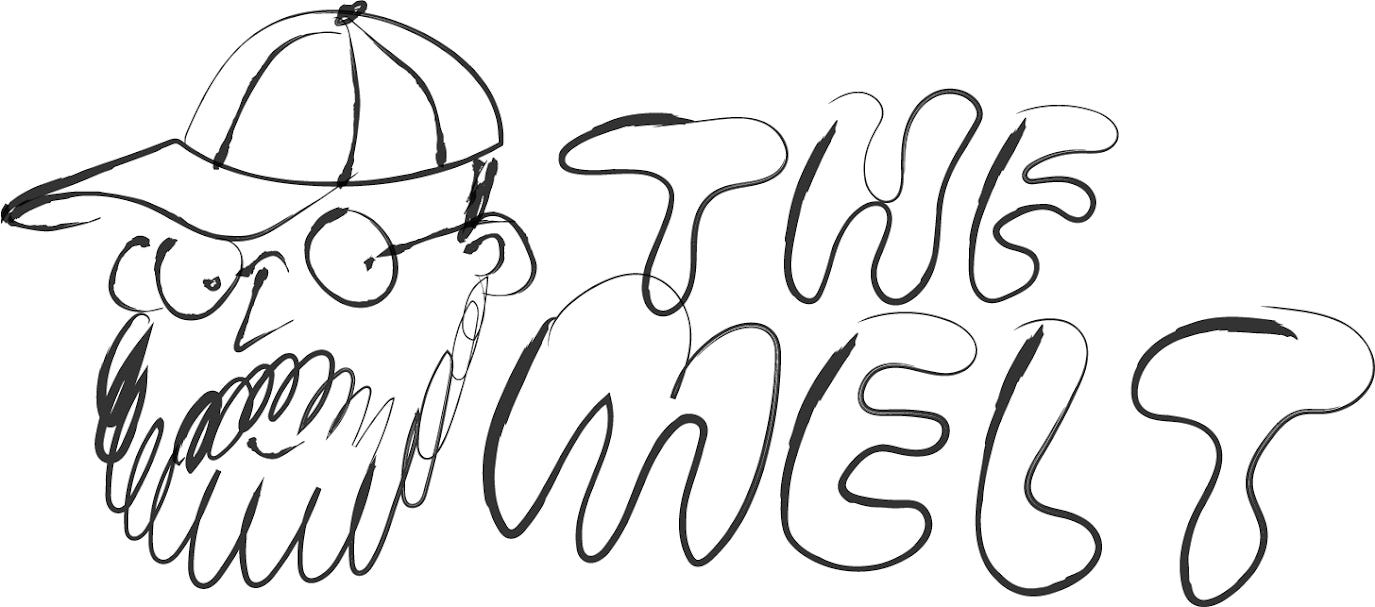The image portrays a graphic design featuring a doodle-style sketch of a man's face on a plain white background. The man is depicted wearing circular glasses, a striped baseball cap with a dot on the top, and has a thick beard that partially obscures his upward-turned mouth, suggesting a smile. Drawn with very thin black ink, the sketch is complemented by text to its right, which reads "THE MELT" in a bubbly, black-outlined font without any interior filling. The entire composition is rendered in black and white, emphasizing the simplicity and starkness of the design.